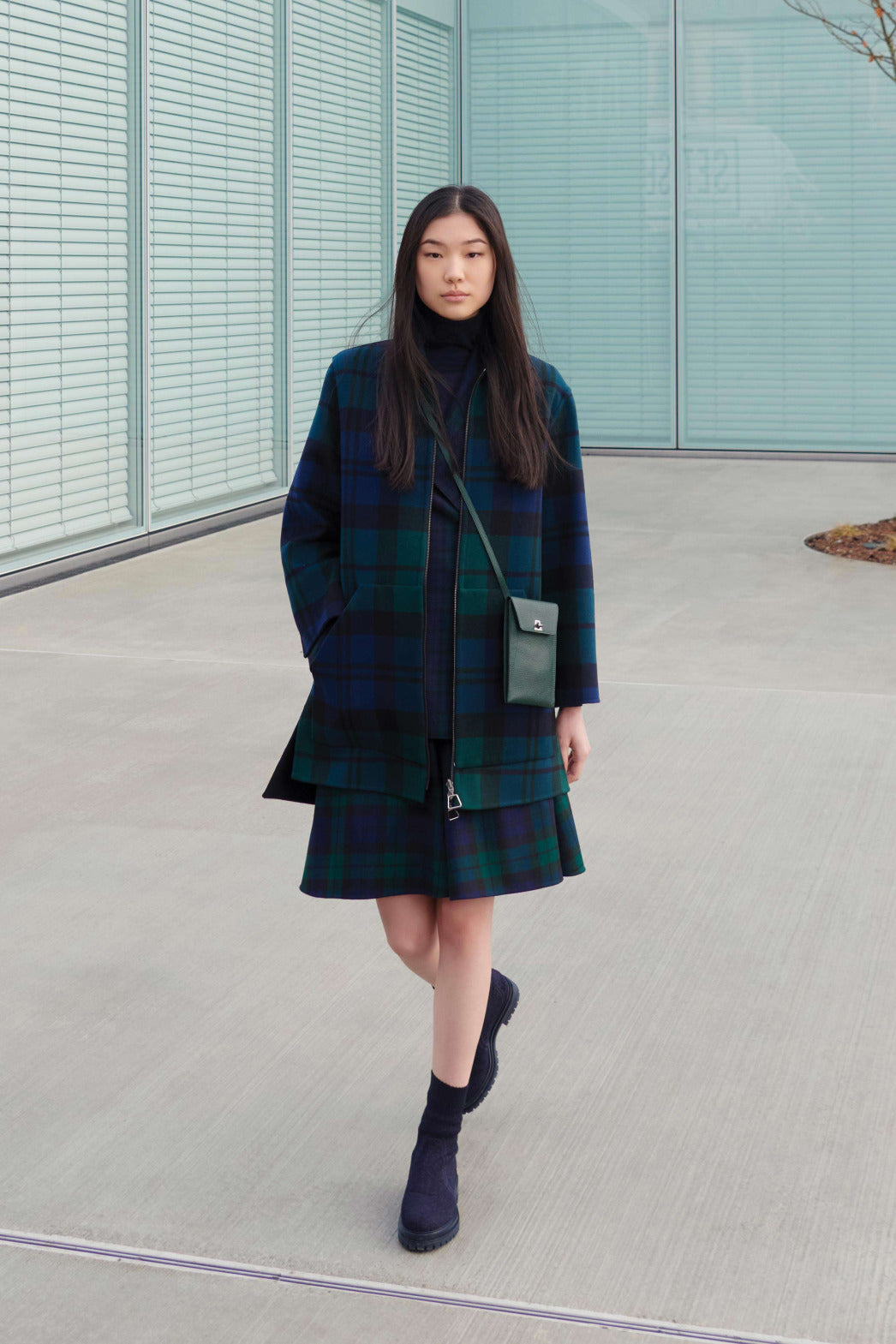The image captures a striking young woman of Asian descent, aged between 15 to 25, with long, straight black hair cascading below her chest. She sports a chic, coordinated outfit featuring a two-tone green and navy blue plaid jacket with large pockets and a flared hem, paired with a matching plaid skirt that reaches just above her knees. Underneath, she wears a dark navy or possibly dark gray shirt. Her ensemble is completed with stylish black ankle booties and a small black purse slung across her shoulder. She is walking across a beige floor, her hand tucked into one jacket pocket while the other hangs by her side, her gaze forward with a serious expression. The background shows green walls resembling blinds, adding an element of ambiguity as to whether she is indoors or outdoors. A large window with closed white blinds and a glimpse of a tree further accentuate the setting.